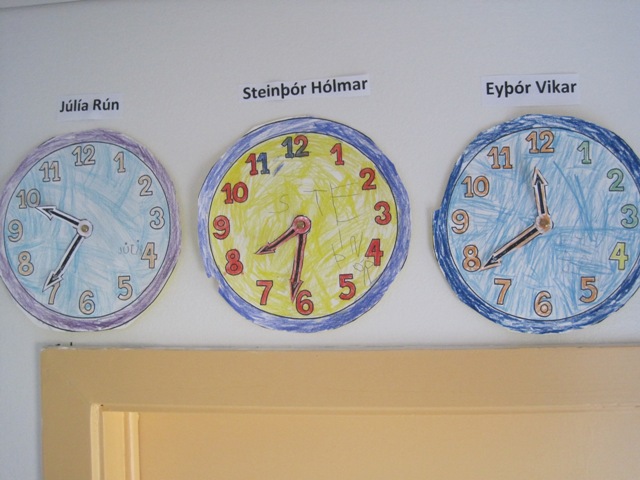Above the doorway, there are three intricately drawn clocks, each accompanied by a label identifying them.

1. The clock on the right features a purple frame with a blue face, adorned with vibrant yellow numbers. Above this clock, a sticker reads, "Julia Run."
   
2. The middle clock has a yellow face and a round base, complemented by red numbers that stand out. Above it, there is a label that says, "STI and BOR HOLMAR."

3. The clock on the left is encased in a round blue frame with a matching blue face. It also features a sticker above it, reading, "EYBOR VIKAR."